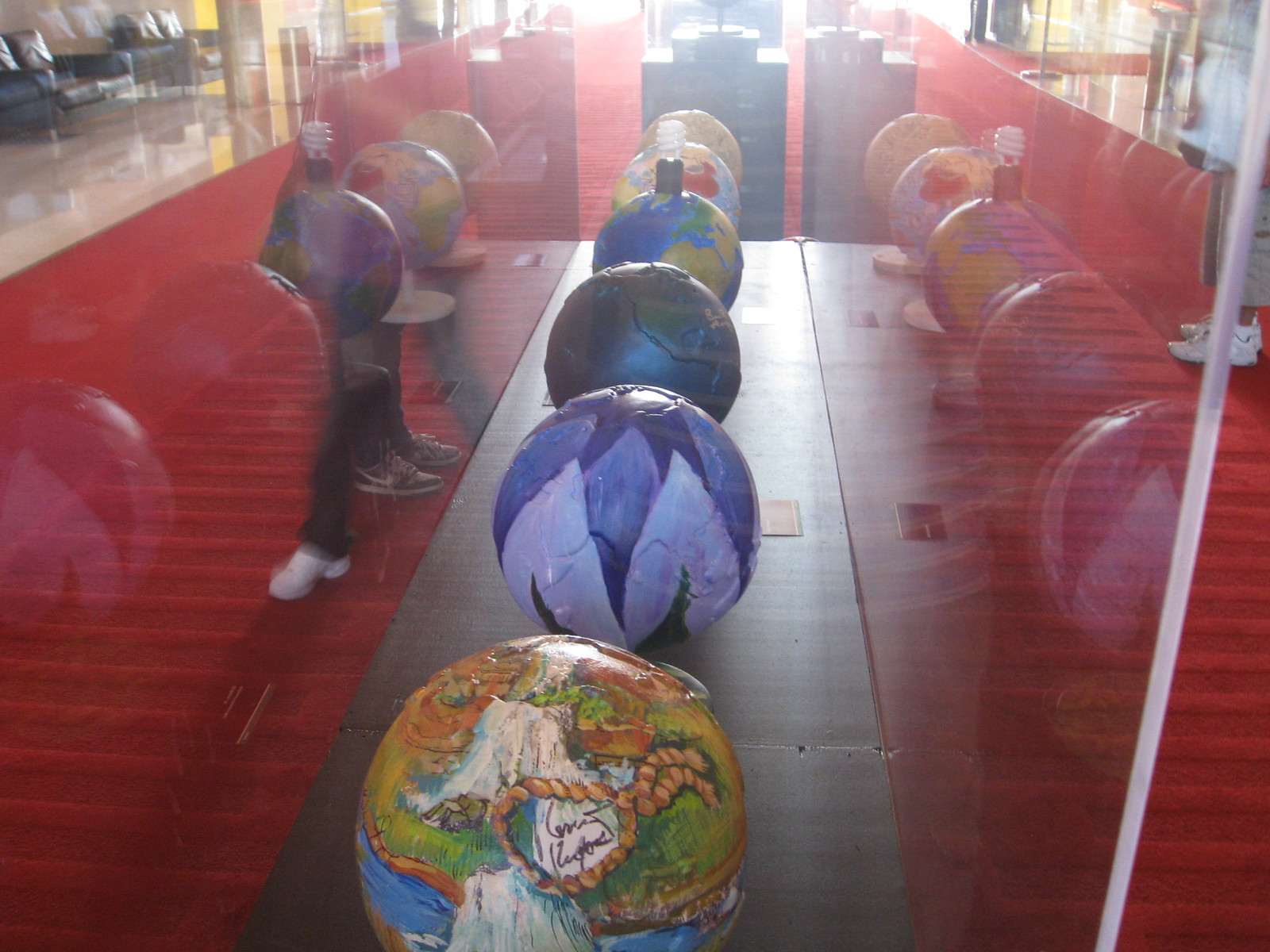Captured within this blurred photograph is an installation at an art exhibit, seemingly taken through a reflective glass or plastic panel, causing the image to be interspersed with both internal and external reflections. The primary focus of the image is a collection of six spherical, globe-like objects encased within a glass container. Each sphere boasts a unique painted design: one flaunts an Earth motif, another displays a purple design with varying shades culminating in a triangle, while yet another showcases a landscape scene. There's also a globe with blue spikes set against a lighter blue background. The remaining spheres, though artistically decorated, are harder to decipher. Positioned beside the glass case is a red carpet, and at least two individuals are nearby, adding to the sense of an open, bustling space such as a train station or library. Red walls border the scene, reflecting the vibrant globes, and a bright morning light from what might be a window illuminates the upper section of the photograph. Additionally, indistinct objects, perhaps couches, are visible in the background, further enhancing the eclectic ambiance of this intriguing art display.